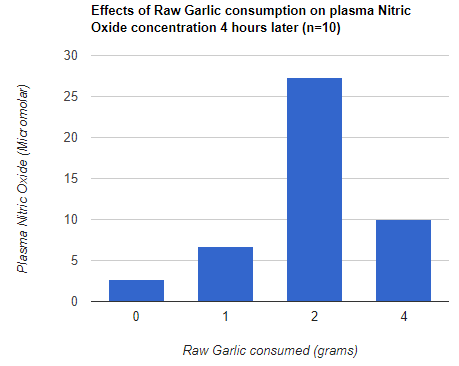This detailed infographic, devoid of any background and set against a white backdrop, presents findings from a scientific study on physiology. The study is titled "Effects of Raw Garlic Consumption on Plasma Nitric Oxide Concentration Four Hours Later (N=10)." The vertical axis of the graph is labeled "Plasma Nitric Oxide (micromolars)" and ranges from 0 to 30 micromolars, in increments of 5. The horizontal axis at the bottom right is labeled "Raw Garlic Consumed (grams)" with measurements at 0, 1, 2, and 4 grams.

The data is illustrated through blue bar graphs for each level of garlic consumption. The bar for 0 grams shows a nitric oxide concentration between 0 and 5 micromolars. For 1 gram of raw garlic consumed, the concentration slightly exceeds 5 micromolars. At 2 grams, the concentration spikes dramatically, falling between 25 and 30 micromolars. However, at 4 grams, the concentration drops back to approximately 10 micromolars. The graph thereby examines and highlights the nuanced impact of varying amounts of raw garlic on nitric oxide levels in blood plasma, suggesting potential nutritional and physiological applications, possibly relevant to sports science and health.